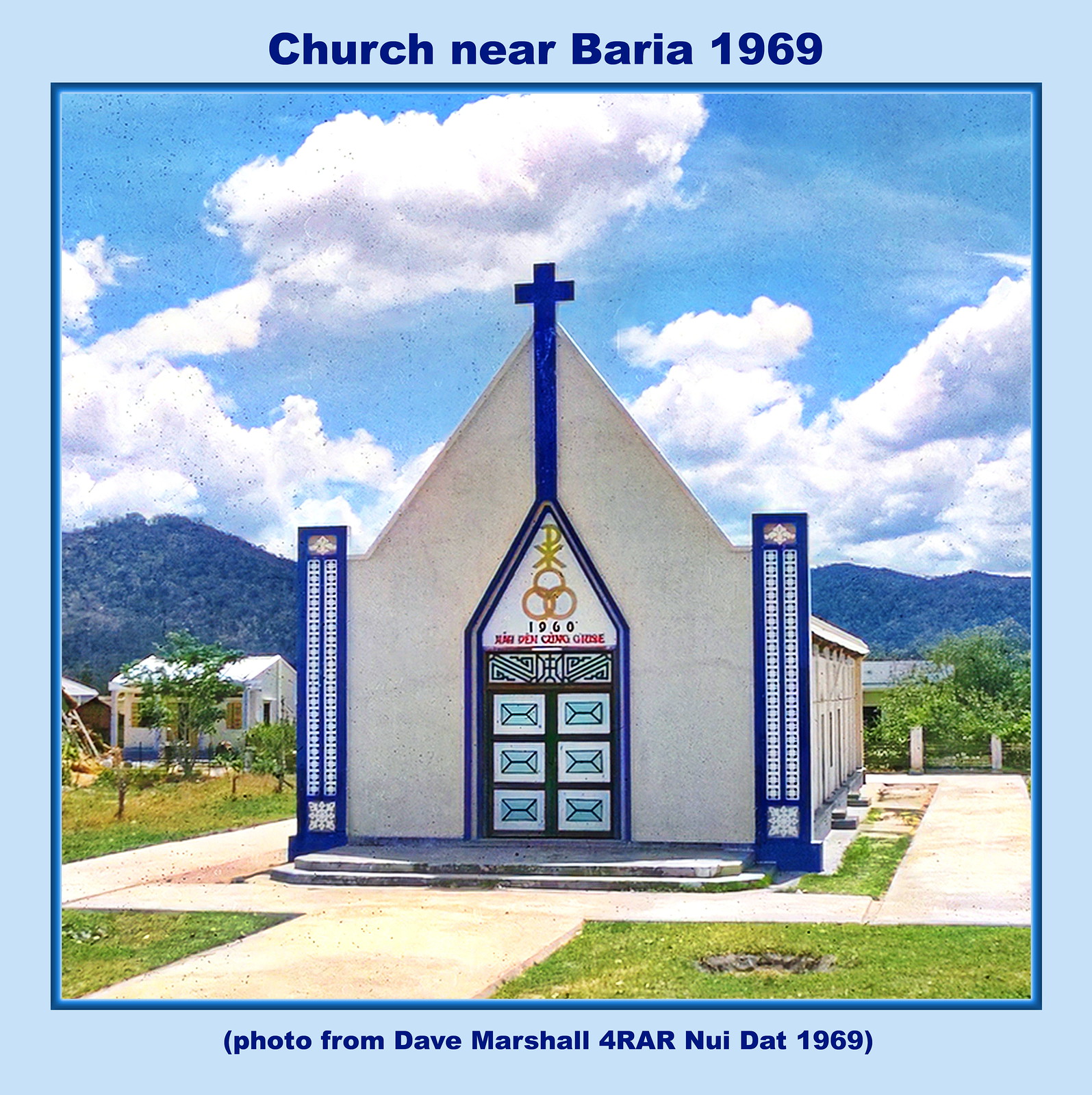A picturesque image from 1969 features a charming, small white and blue church near Berea, nestled under a vibrant blue sky filled with puffy white clouds and backed by rolling, tree-covered mountains. The church exterior is adorned with a striking blue cross that extends past the roofline, along with intricately designed, blue and white pillars on either side of the ornate front doors—these pillars bear snowflake-like patterns. Surrounding the church is a cement walkway and green patches of lawn, leading to different perspectives of the building. In the background, several houses and a variety of trees populate the landscape, showing a tranquil setting. The photograph itself is framed with a light blue border, with “Church near Berea, 1969” inscribed at the top, and “Photo from Dave Marshall for RAR, Nui, 1969” written at the bottom. The church's main door, prominently tall with a rectangular base and various religious symbols, adds to the striking detail of this serene and historical scene.